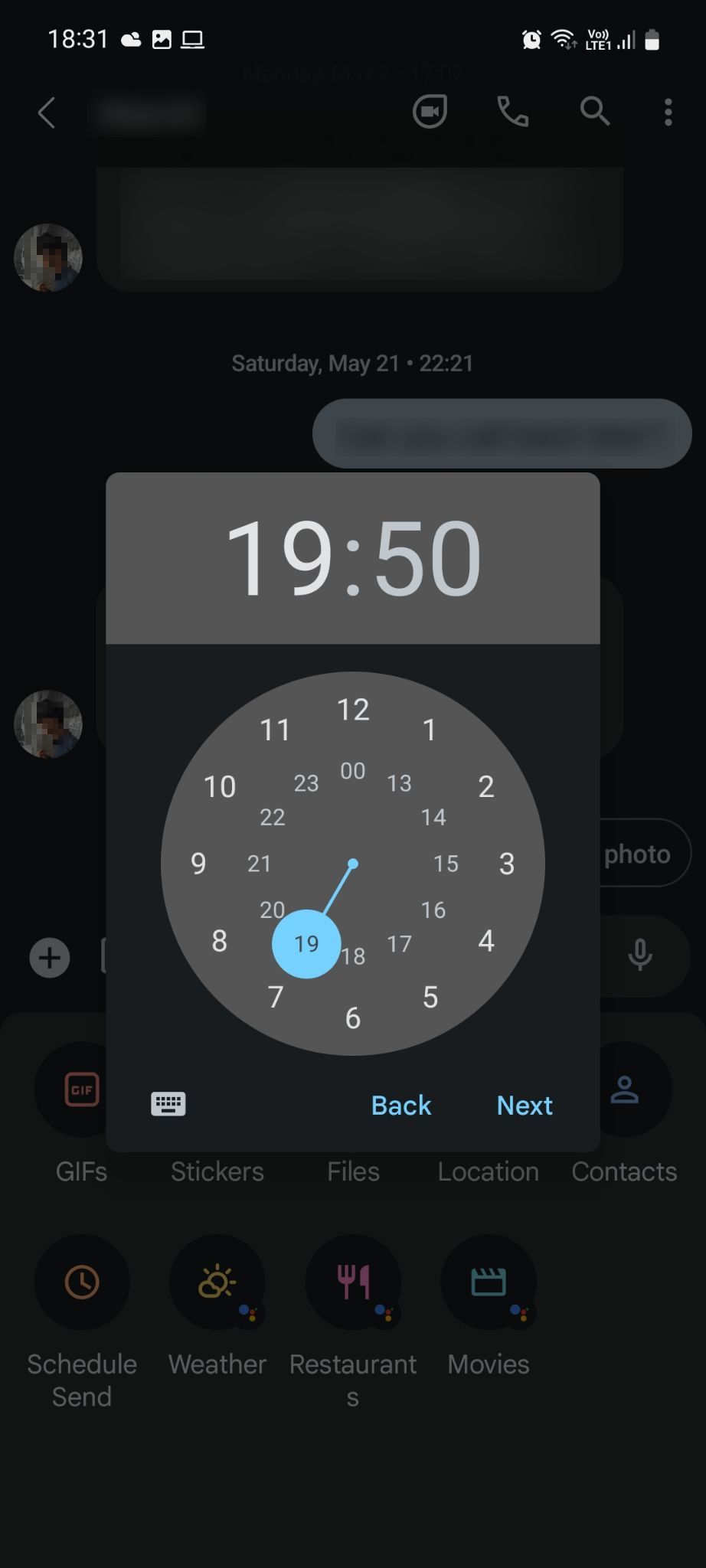This screenshot captures the time picker interface of a mobile phone's messaging app, set in a dark theme. The interface prominently displays a clock face set to 19:50, with the hour hand pointing to 19 and the minute hand pointing to 50. Above the time picker, a timestamp reads "Saturday, May 21st, 2221," marking the date of the last received message. The blurred background offers a glimpse of the chat interface, including a partially obscured profile picture of the recipient. The background's theme features shades of gray and black.

From the interface, you can see various functionality icons such as gifts, stickers, files, location, contacts, schedule send, weather, restaurants, and movies. There's an additional timestamp showing "18:31" within the blurred conversation. At the top of the screen, status indicators display a Wi-Fi signal, LTE connectivity, and battery life, though these are partially obscured. Overall, the screenshot provides a detailed view of the app's robust scheduling features within the dark-themed time picker interface.